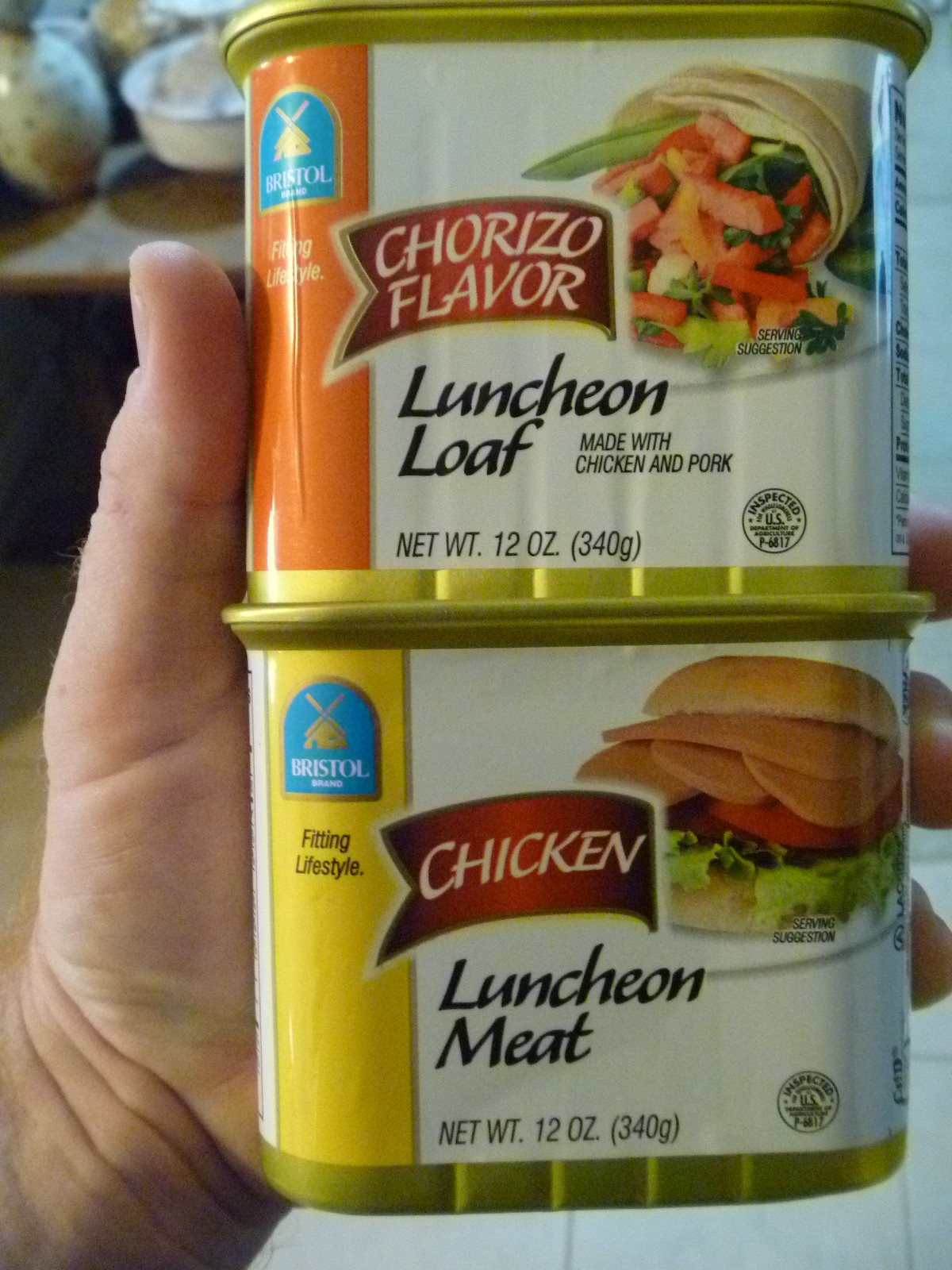The image depicts a left hand, presumed to be that of a fair-skinned man, holding two vertically stacked, 12-ounce cans of luncheon meat in a first-person POV style photo. The scene is set in what appears to be a kitchen, with glimpses of white tile flooring and a wooden countertop in the background, though the cans and hand occupy most of the frame. The top can, featuring an orange label, is Bristol brand chorizo flavor luncheon loaf made with chicken and pork. The label prominently displays text reading "Fitting Lifestyle" and an image of a wrap overflowing with ingredients like lettuce, vegetables, and meat. Below it, the yellow-labeled can reads Bristol brand chicken luncheon meat, illustrated with a sandwich filled with chicken, lettuce, and tomato. Both cans bear similar branding elements and emphasize their respective flavors and uses through vivid imagery and detailed descriptions.